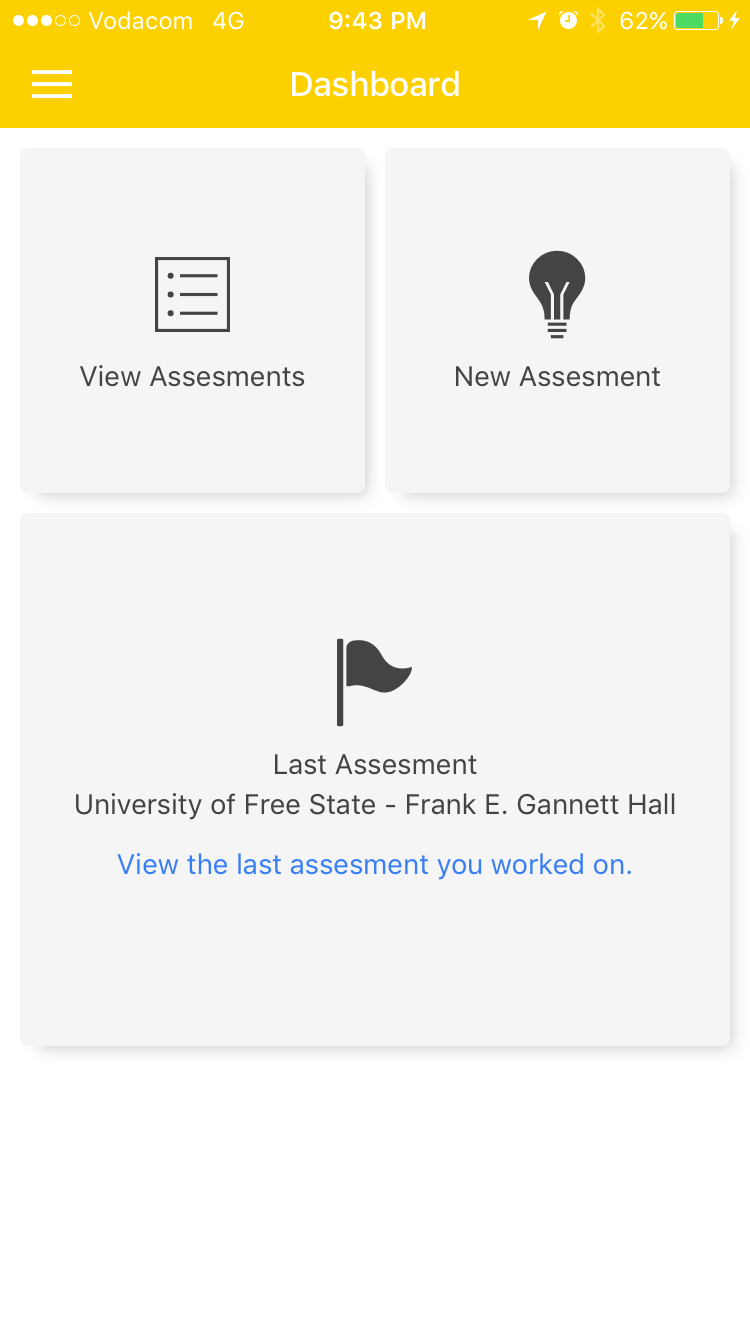This image is a vertical screenshot from a mobile device, prominently featuring a bright yellow banner at the top edge. The rest of the screenshot has a clean white background, framed by minimal borders on the left, right, and bottom edges. At the very top, the status bar indicates a Vodacom 4G network connection in the upper left-hand corner, with three out of five signal dots filled. There are also three vertical lines on the left-hand side, indicating a menu.

Centered at the top, the time is displayed as 9:43, directly above the word "Dashboard". On the upper right-hand corner are several icons, including a battery icon showing a 62% charge in green.

Beneath the status bar, two square pop-up boxes are aligned horizontally. The left box, labeled "View Assessments", features an icon consisting of a square with three dots and three lines. To the right, a gray light bulb icon accompanies the text "A New Assessment".

The largest pop-up box is located at the bottom and contains a gray flag icon. This box is labeled "Last Assessment" with additional details: University of Free State, Frank E. Gannett Hall. A blue text link below reads “View the last assessment you worked on.” This link is designed to provide quick access to the most recent assessment activity.

In summary, this detailed mobile screenshot showcases a user dashboard with essential status indicators, navigation options for viewing and starting new assessments, and a direct link to the most recently accessed assessment.